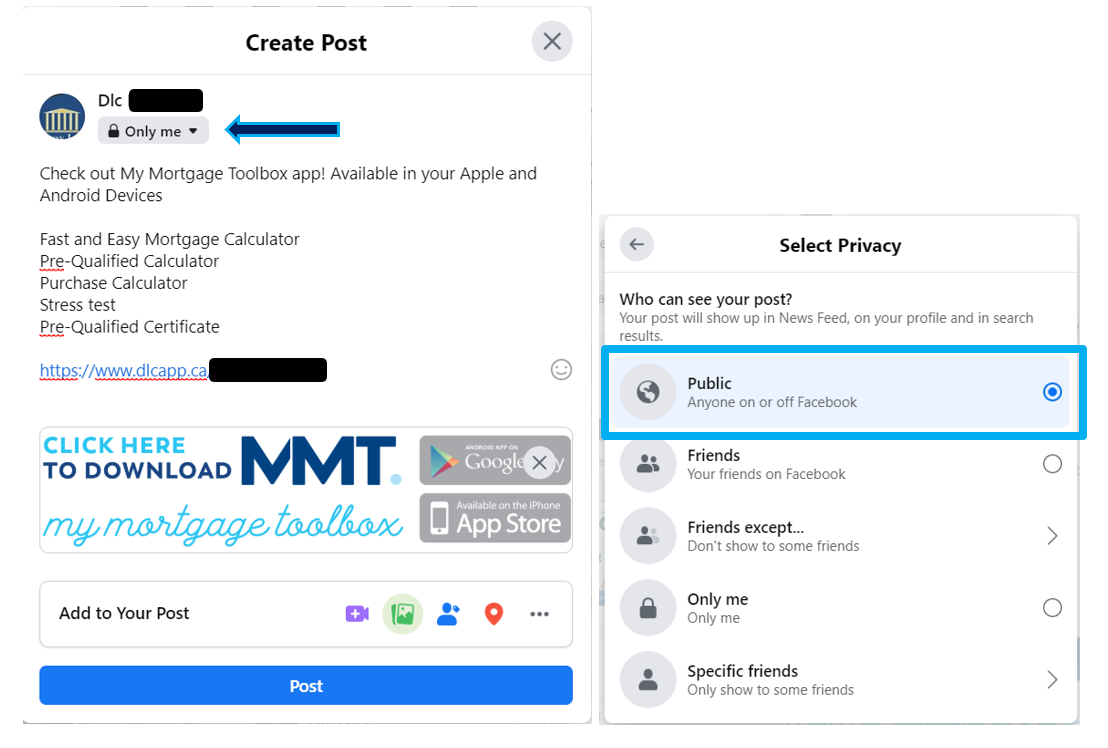This image is a detailed screenshot of an interface with two distinct sections. The left section, titled "Create Post," appears to be from a DLC-branded application. The title includes partially redacted text, suggesting some privacy considerations. Below the title, there's a button labeled "Only Me" accompanied by a lock icon, and a navy blue arrow points to this button, indicating a potential instruction or guidance.

Following this, a line of text promotes a mortgage tool application, highlighting its availability on both Apple and Android devices. The features of the app are listed, including a fast and easy mortgage calculator, a pre-qualification calculator, a purchase calculator, a pre-qualified certificate, and a stress test. There's a partially redacted URL at the bottom (dlcapp.ca), likely leading to more resources.

Immediately below, there's a banner from MT, featuring a call to action in blue text: "Click to download my Mortgage Toolbox." To the right of this banner are two gray buttons for downloading the app from the Google Play Store and the Apple App Store.

At the bottom of this section is a rectangular input field labeled "Add your post," flanked on the right by three icons: a red location icon, a blue silhouette of a person, and a purple camera button. Below these, a blue "Post" button is prominently displayed.

The right section, titled "Select Privacy," outlines who can see your post with five options. The currently selected option is "Public," highlighted in a blue box with a globe icon, indicating accessibility to anyone on or off Facebook. The other options include "Friends" (two silhouettes), "Friends except…" (two silhouettes with one grayed out), "Only me" (lock icon), and "Specific friends" (one silhouette). Each option is represented with corresponding icons for easy identification.

This screenshot appears to be part of a social media or app interface designed for creating and sharing posts, with detailed privacy settings and promotional content for a mortgage tool.